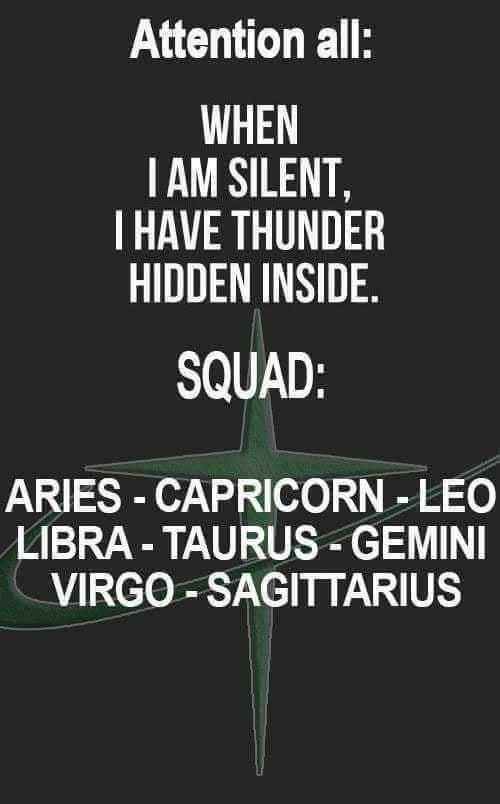This image features a text overlay on a black background. The text is written in white, using a plain, bold font that resembles Arial. It starts with the words "Attention all" in lowercase, followed by capitalized text that reads: "WHEN I AM SILENT, I HAVE THUNDER HIDDEN INSIDE. SQUAD: ARIES, CAPRICORN, LEO, LIBRA, TAURUS, GEMINI, VIRGO, SAGITTARIUS." The text is centered on the image, creating a clear and balanced layout. 

In the background, there is a subtle, green design that combines elements of a stylized cross and a thin line resembling a Nike swoosh. This design is located towards the center bottom of the image. The cross-like shape is not a traditional crucifix; it has a more abstract and star-like appearance. The combination of the bold, white text and the black background, with the green design elements subtly visible behind the text, gives the image a striking and modern aesthetic, reminiscent of a digital poster or ad.